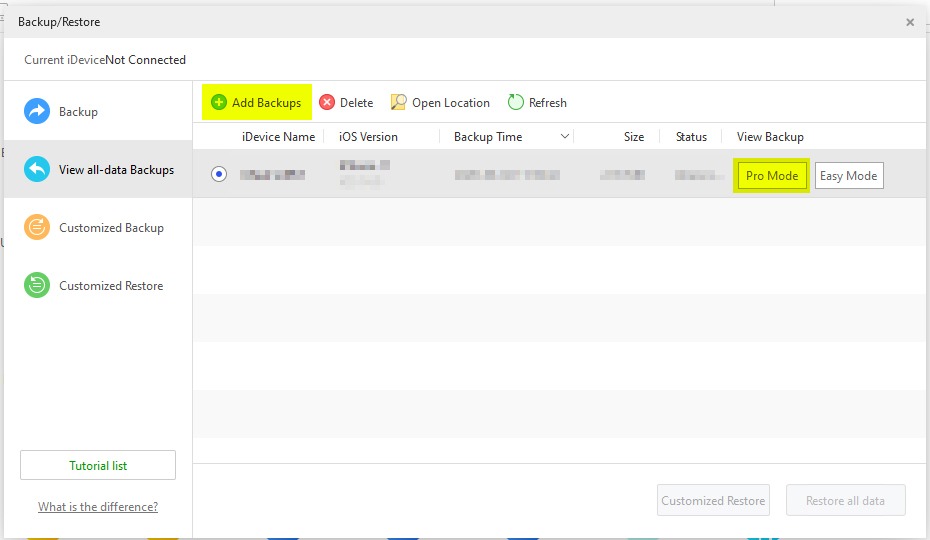Here is a cleaned-up and detailed caption for the image:

---

The image displays a computer screen showing a user interface for a data management application. At the top left, there are buttons labeled "Backup" and "Restore." Directly below, it says "Current iDevice: Not Connected." The left sidebar contains four categories: "Backup," "View All Data Backups," "Customize Backup," and "Customize Restore." At the bottom of this sidebar, there is an option labeled "Tutorial List."

On the right-hand side, the upper section features four clickable categories: "Add Backups," highlighted in yellow with a green circle and a plus sign next to it, alongside "Delete," "Open Location," and "Refresh." The main section has a table with column headers: "Device Name," "iOS Version," "Backup Time," "Size," "Status," and "View Backup." The details under the first five columns are blurred out. The "View Backup" column has two options: "Pro Mode," highlighted in yellow, and "Easy Mode," displayed as a white box.

The lower part of the screen has alternating light gray and white horizontal stripes as the background. In the bottom-right corner, there are two non-interactive options: "Customize Restore" and "Restore All Data."

---